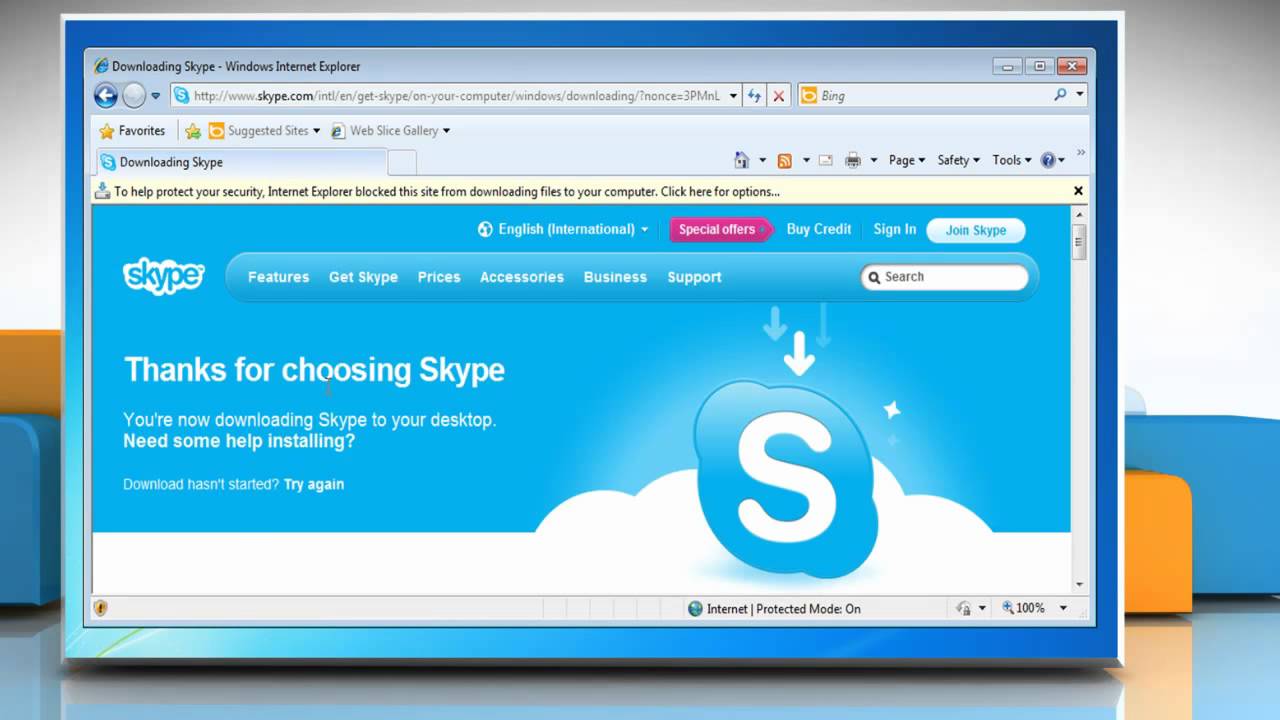The screenshot captures the monitor during a visit to the Skype website, as displayed in Windows Internet Explorer. The browser header is light blue, featuring tabs for "Favorites," "Suggested Sites," and "Web Slice Gallery," with the address bar showing "Skype.com." In the upper-left corner, dark blue text reads “Downloading Skype, Windows Internet Explorer.”

Dominating the bottom two-thirds of the screen is a light blue background resembling the sky, complete with a cloud graphic at the lower edge. Prominently placed in the upper left of this sky-themed section is the Skype logo, rendered in blue text and flanked by white clouds.

A horizontally aligned menu spans the page from left to right, listing the options: Features, Get Skype, Prices, Accessories, Business, and Support. Adjacent to the menu, a white search bar sits neatly to the right. Beneath the navigation menu, bold white text proclaims, "Thanks for choosing Skype," followed by a message indicating that the Skype download to the user's desktop has commenced.